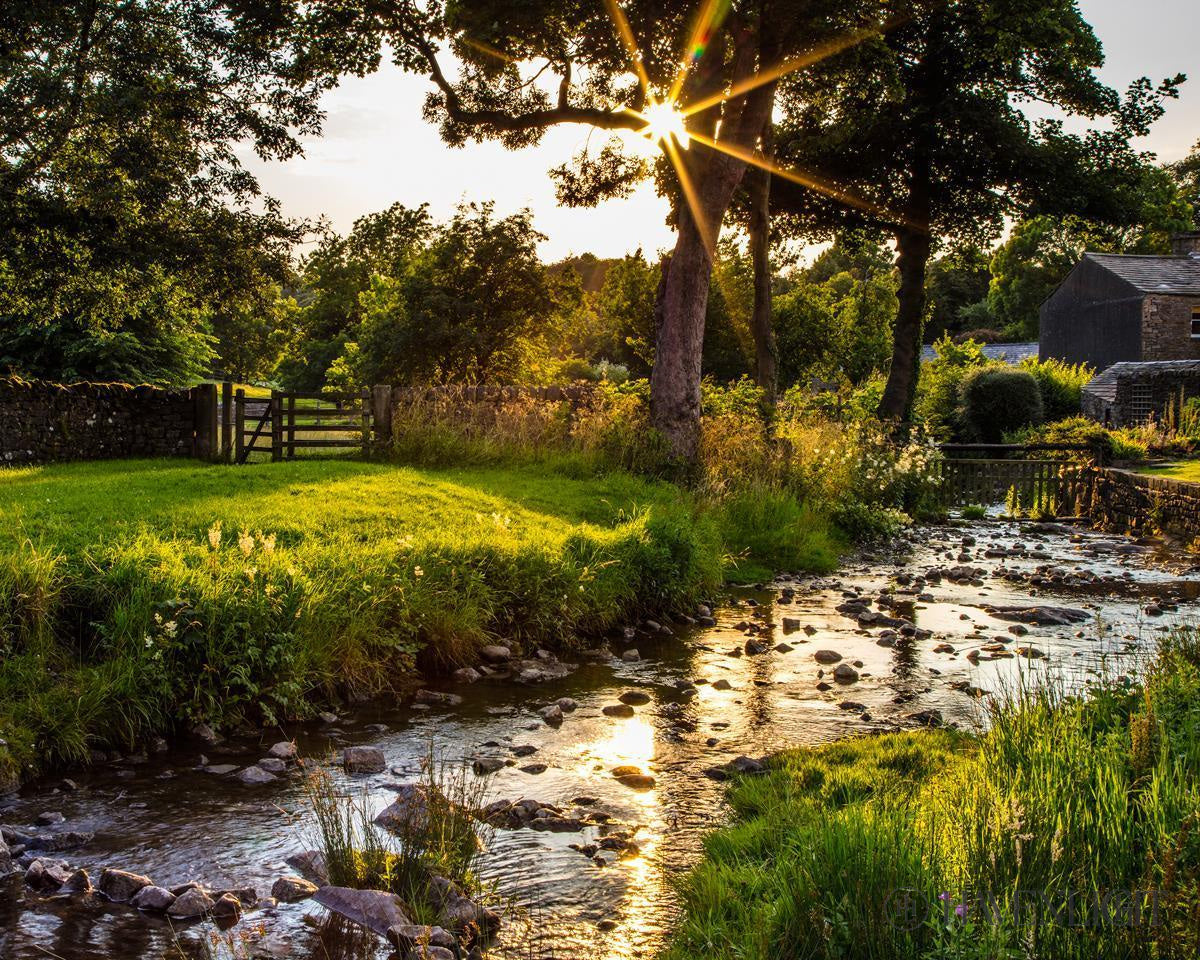A picturesque country house nestles in the serene landscape, positioned in the top right middle of the photograph. The house is set beside a collection of trees, which extend towards the left and downwards, creating a lush backdrop. Dominating the foreground, a tranquil creek flows from the bottom left corner, meandering towards the right middle. The water is calm, punctuated by stones and bordered by grassy embankments raised about three to four feet above the surface. The grass and bushes on either side are rich green, highlighted by patches of white flowers and lime-green hues, complemented by a scattering of foliage.

A charming brown picket fence spans the mid-distance of the image, and in front of it lies a verdant grassy area. Beyond this, a rustic stack of wood adds to the rural charm. The scene is bathed in the warm, rich light of a setting sun, casting a lightish yellowish orange glow, which streams through the branches of a large tree in the somewhat foreground on the opposite side of the creek. The sky above is a pale white, gradually transitioning to deeper colors as the sun nears the horizon. Ripples in the water reflect the sunlight, adding a shimmering effect to the serene creek, where stones break the surface intermittently. The entire composition is framed by a busy tree line in the distance, completing this idyllic country setting.